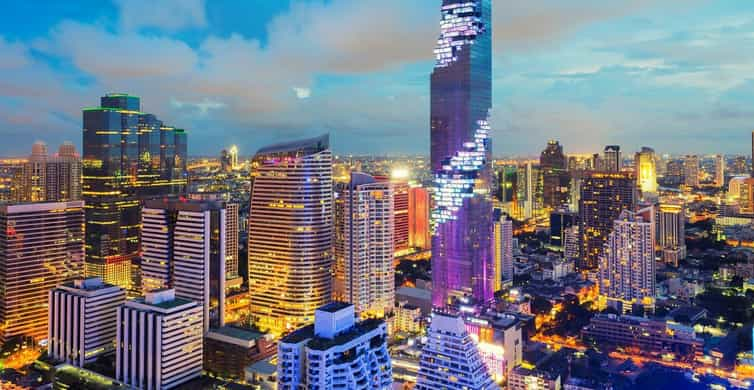This image presents a breathtaking aerial view of a bustling city, possibly Tokyo or Singapore, taken from a drone or helicopter during dusk. Dominating the skyline is a towering skyscraper, bathed in a striking purple light that reaches close to the edge of the frame. Surrounding this central high-rise is a cluster of smaller buildings, similarly aglow with purplish hues, creating a vibrant, illuminated mosaic. Sprinkled among these structures are buildings emitting a cool blue and green light, adding to the city's ethereal ambiance.

The foreground reveals a tangle of city streets, busy with cars and pedestrians, though the time of day suggests it should be less illuminated. This unexpected brightness accentuates the dense urban fabric, which only allows sporadic glimpses of trees and green spaces. The sky above transitions from a clear blue on the left to a cloudy, bluish-gray toward the right, encapsulating the city's dynamic energy under the canopy of an impending twilight.